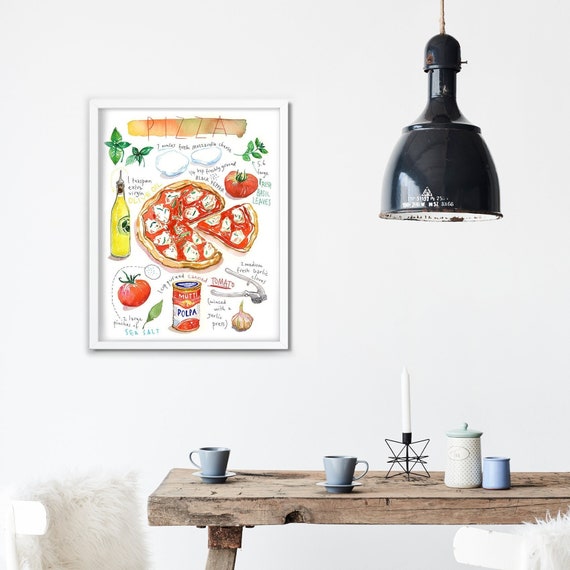The photograph captures a cozy, rustic dining room scene. In the foreground, a brown, rustic wooden table is scattered with three gray-blue mugs, spread out around a decorative metal star holding a white candle. Nearby, there's a glass or ceramic sugar jar with a distinctive green top. The table is flanked by two white, plush chairs covered in a fabric mimicking white fur. Above the table, a black, cone-shaped dome light hangs from the ceiling, illuminating the setting. The background features a plain white wall adorned with a framed, hand-drawn-style image showcasing various pizza ingredients such as tomatoes, garlic, olive oil, and cheese, with a pizza and a slice prominently displayed in the center. The frame is simple and white, seamlessly blending with the wall. The entire scene is bathed in natural light, lending a warm and inviting atmosphere.